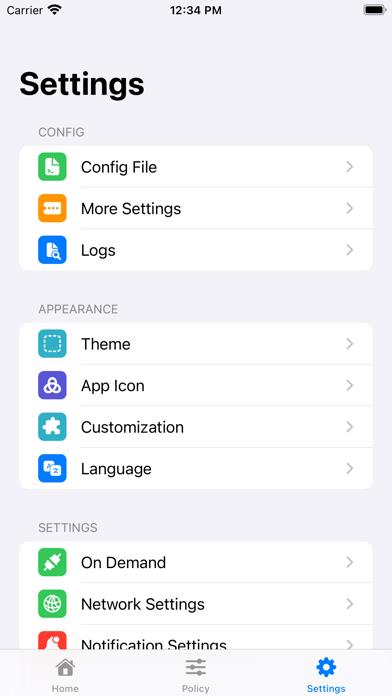This detailed screenshot captures a glimpse of a mobile device's settings menu. At the top, the carrier name is displayed in black font, and a strong Wi-Fi signal icon is prominently visible. The screenshot was taken at 12:34 p.m., as indicated by the time on the status bar. The battery icon on the right shows a full charge. The overarching menu title "Settings" is bolded in large black font against a white to whitish-gray background.

Within the settings menu, several options are listed:
1. **"Config"**: Displayed in gray with a green box, accompanied by a caret indicating it can be expanded.
2. **"More settings"**: Highlighted in an orange box with white text.
3. **"Logs"**: Contained in a blue box with a magnifying glass icon next to it.
4. **"Appearance for theme"**: Shown in a blue box.
5. **"App Icon"**: Also displayed within a blue box.
6. **"Customization"**: Featured in a green box.
7. **"Language"**: Indicated with an A to Z representation.
8. **"Settings for on-demand"**: Enclosed in a green box.
9. **"Network settings"**: Presented in a green box.
10. **"Notification settings"**: Highlighted in a red box.

The caption concludes with a courteous "Thank you for watching."